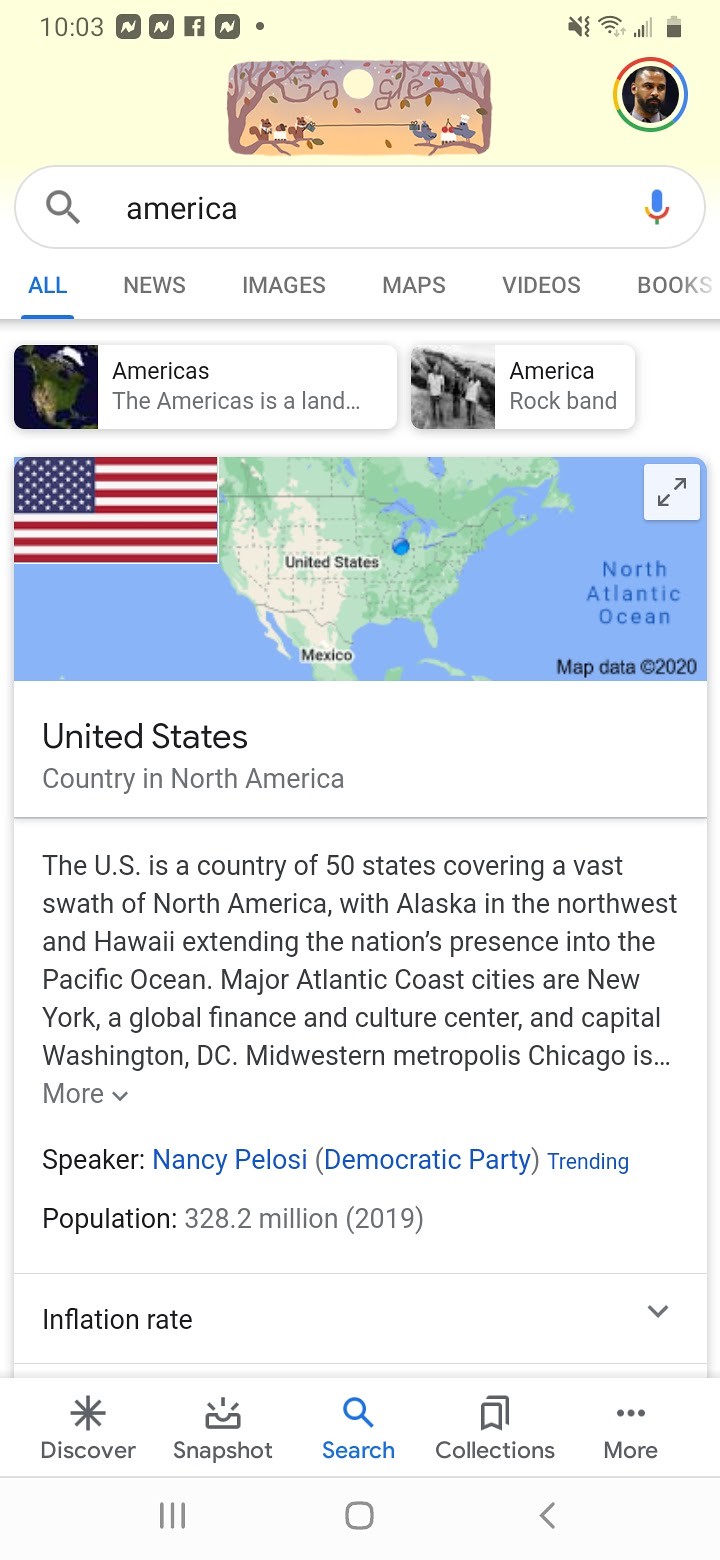**Detail-Rich Caption:**

The screenshot captures the results of a Google search for "America" on a smartphone. At the top, the screen displays a header labeled "Americas," accompanied by a map image of the continent. In the top left corner, the U.S. flag is prominently displayed. Beneath the flag, the text reads, "United States, country in North America," followed by demographic information, "Population: 328.2 million (2019)." 

Prominent below this data, there's mention of Nancy Pelosi as the Speaker from the Democratic Party. Also noted is a brief reference to the inflation rate, though specifics are missing.

Towards the bottom of the screen is the navigation menu with icons labeled: Discover, Snapshot, Search, Collections, and an option labeled 'More', represented with three vertical dots. Additional text provides a brief overview of the country: "The U.S. is a country of 50 states covering a vast swath of North America with Alaska in the northwest and Hawaii extending the nation's presence into the Pacific Ocean."